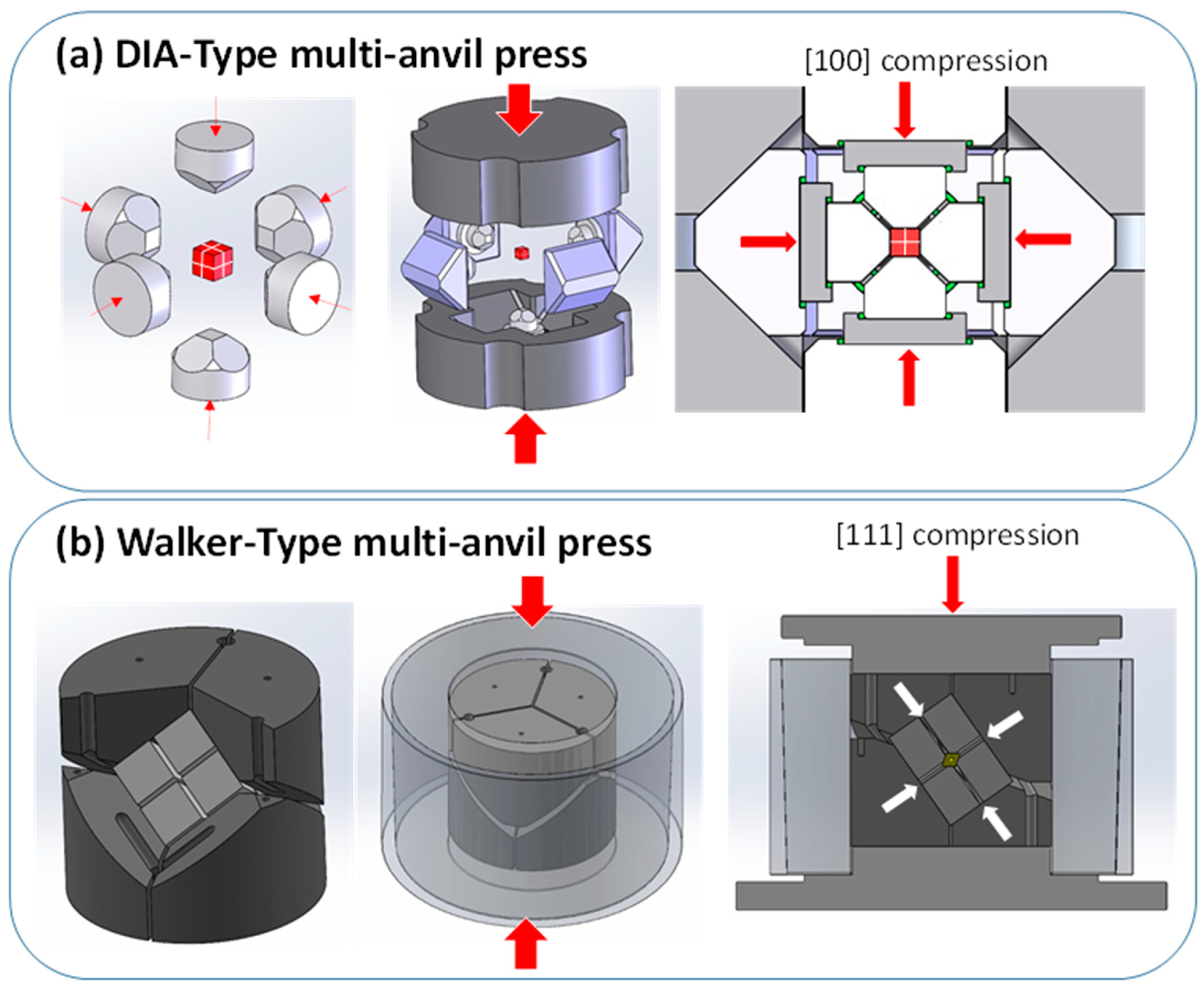The instructional image delineates the assembly and functionality of a DIA type multi-anvil press through a series of detailed diagrams. The top section, labeled "DIA type multi-anvil press," comprises three primary images. The first image illustrates the disassembled parts, including distinctive silver octagonal components. The central image showcases the partial assembly with two gray cylinders, highlighted by red arrows indicating directional compression from the top and bottom. Here, an internal view depicts complex triangular configurations, emphasizing 100 compression points. The final image on the right shows the fully assembled press, complete with additional red arrows to demonstrate the flow and mechanism of compression. 

The bottom section, labeled "Walker type multi-anvil press," similarly contains three images. The initial image portrays the base circular cylinder object. The middle image presents a clear object encasing a cylinder, showing further stages of assembly. The concluding image displays a dark gray, boxy unit, potentially a functional installation resembling a silver oven, with arrows signifying internal compression dynamics and unit operation pathways. The detailed red and gray diagrams, with explicit arrow indicators, carefully illustrate the assembly, internal workings, and final installation of both multi-anvil press types.